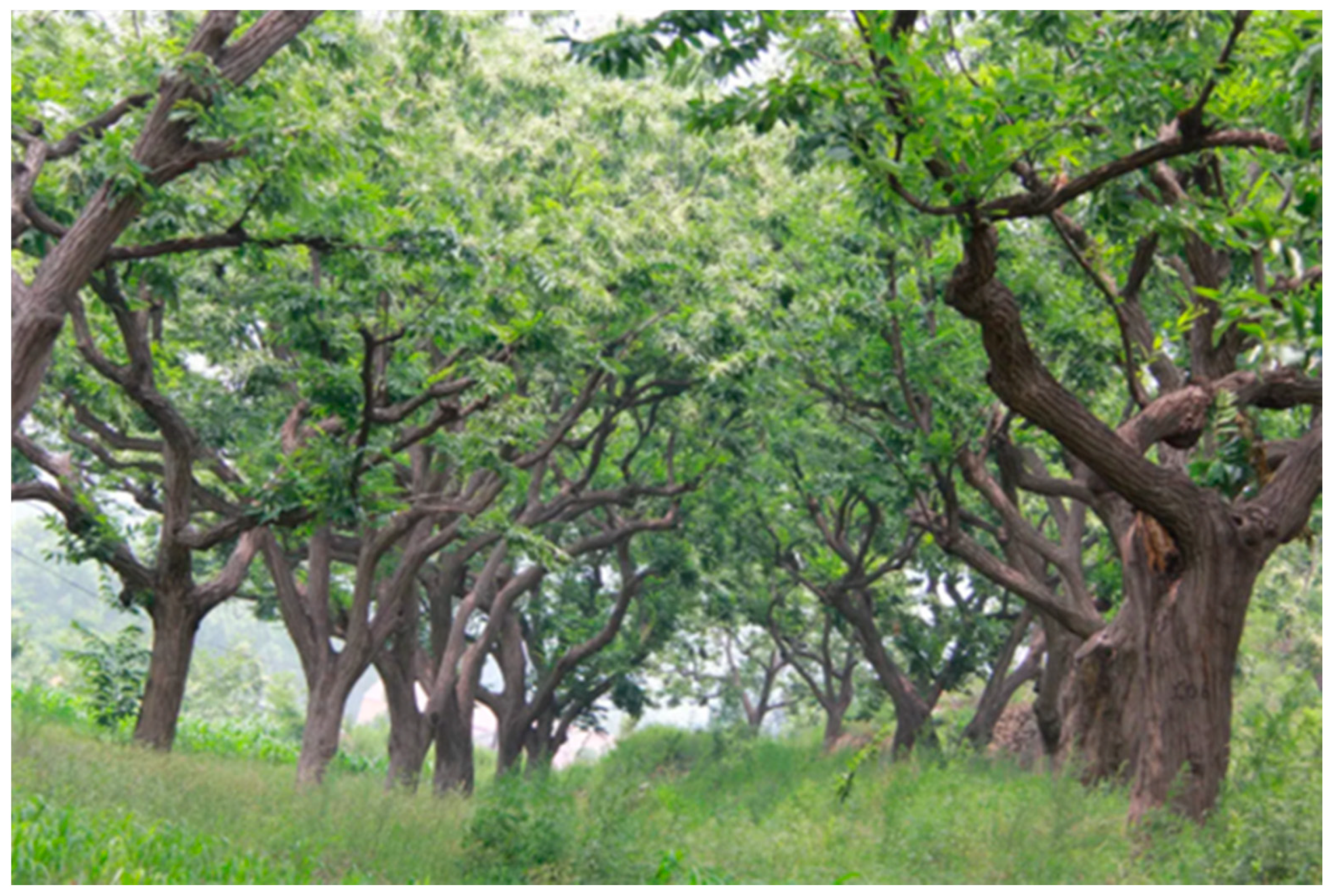The image depicts a slightly blurry and skewed outdoor scene dominated by tall grass and a variety of trees. The setting appears to be a sunny day. Trees are arranged in two somewhat irregular rows on both the left and right sides of the field. The trees have long trunks that branch out into thicker limbs, creating a mixed canopy of lush green leaves, with some white flowers visible at their tops. As the branches extend into the sky, they intertwine, forming a tunnel-like arch. The background shows additional trees at a considerable distance, adding depth to the scene. At the lower left side of the image, a power line can be faintly detected through the grassy expanse. The predominant colors in the image are various shades of green and brown.